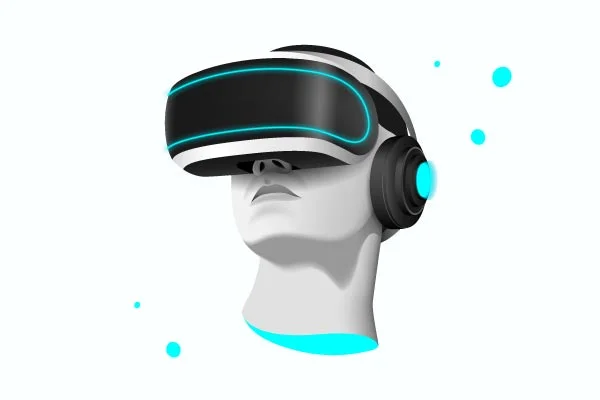The image depicts a stylized drawing or AI-generated representation of a mannequin head floating against a white background. The mannequin head, shaded in a grayish tone, is adorned with a pair of advanced, futuristic glasses covering its eyes and part of its nose. The glasses feature a black visor outlined by a neon turquoise line in an oval shape. In addition, the head wears a gray headband connected to black earphones that display a neon turquoise light at the center. The neck of the mannequin appears to be neatly cut off, revealing an inner glow that is neon turquoise, accentuating the futuristic theme. Surrounding the head are floating neon turquoise bubbles, further enhancing the high-tech, virtual reality aesthetic. The head is slightly turned to the left, tilted upwards, allowing a view of the nostrils and lips from below, adding to the stylized, possibly female appearance suitable for an icon or advertisement.